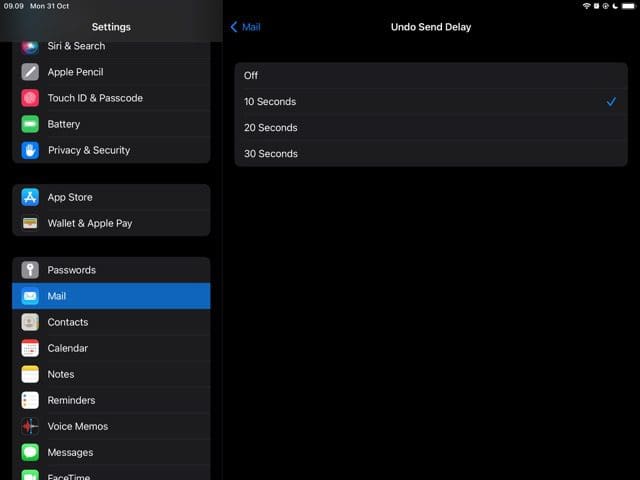The image showcases a digital interface with a black background, likely a settings page on an Apple device such as an iPhone or iPad. The page is dated Monday, 31st October. On the left side, there's a categorized list of navigational options, including:

- Siri and Search
- Apple Pencil
- Touch ID and Passcode
- Battery
- Privacy and Security
- App Store
- Wallet and Apple Pay
- Passwords
- Mail
- Contacts
- Calendar
- Notes
- Reminders
- Voice Memos
- Messages
- FaceTime

Among these options, 'Mail' is highlighted, indicating the current selection. At the top of the highlighted 'Mail' section, the setting "Undo Send Delay" is displayed, with options to set the delay to Off, 10 seconds, 20 seconds, or 30 seconds. The presence of a Wi-Fi icon indicates that the device is connected to a wireless network. Overall, the image seems to depict a settings menu designed for user navigation and customization on an Apple mobile device.